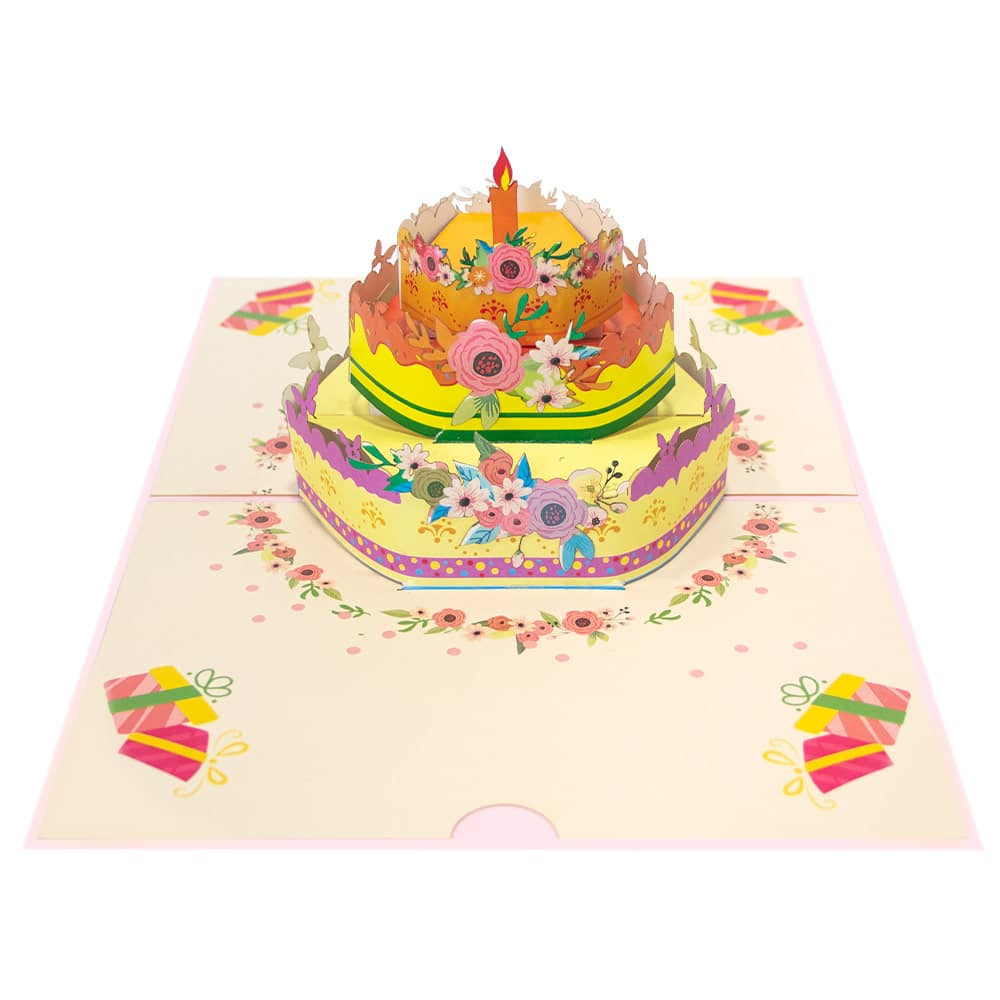This is a detailed concept drawing of a multi-tiered birthday cake, set on an off-white mat with decorative accents. The corners of the mat each feature two intricately drawn presents in different colors, such as pink, yellow, green, and shades of orange, with delicate bows on top. The central focus of the drawing is a three-tiered cake, encircled by a floral wreath. The bottom tier of the cake is light yellow with intricate purple adornments and a variety of flowers in pink, purple, and green at the front. The middle tier is colored yellow with green lines and is also decorated with pink, white, and additional floral patterns. The top tier is orange, embellished with red decals and a garland of pink, white, and orange flowers, crowned by a single prominent orange candle with a red and yellow flame. A purple strip with yellow, blue, and red spots encircles the base of the cake, complementing the overall vibrant design. The mat beneath the cake and presents appears slightly pink in some areas, adding a subtle backdrop that highlights the colorful details of the objects on it.